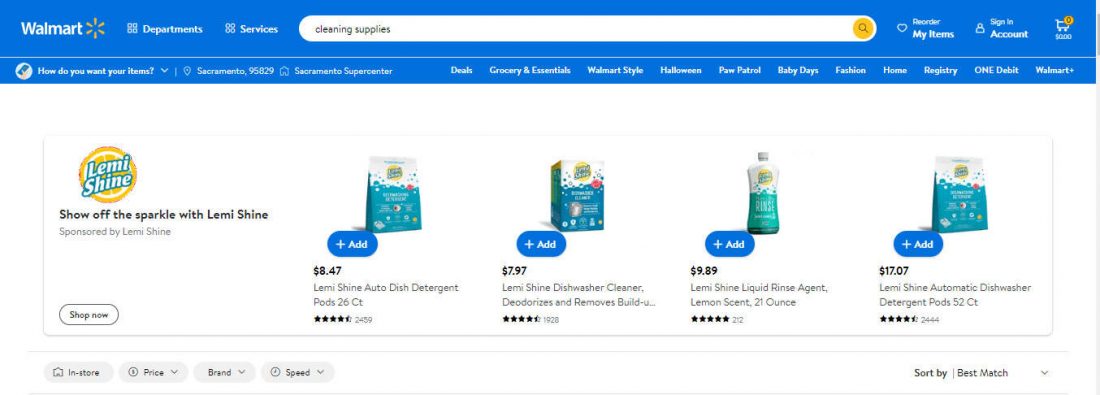This is a landing page from Walmart, characterized by its signature bright blue header. At the top of the screen is a prominent ribbon banner, with "Walmart" displayed in bold white text on the upper left-hand corner, accompanied by the iconic orange Walmart starburst logo. On the right side of the banner, the words "Departments" and "Services" are presented in very small white text. Below the ribbon is a long, white search bar displaying the text "cleaning supplies" in black. Adjacent to the search bar are options reading "Reorder My Items" and "Sign In To Account," followed by a shopping cart icon. The shopping cart icon features an orange circle with a zero inside, indicating no items have been added yet.

Below this, on a clean white background, four different cleaning products are showcased from left to right. In the corner of this section, the brand "LemiShine" is displayed in bold white text with a green outline, positioned over a graphic resembling half of a lemon slice. Directly below, the tagline reads, "Show Off the Sparkle with LemiShine" in black text. Each of the four LemiShine products shown has an image, price, rating indicated by stars, and a blue "Add" button for easy addition to the shopping cart.